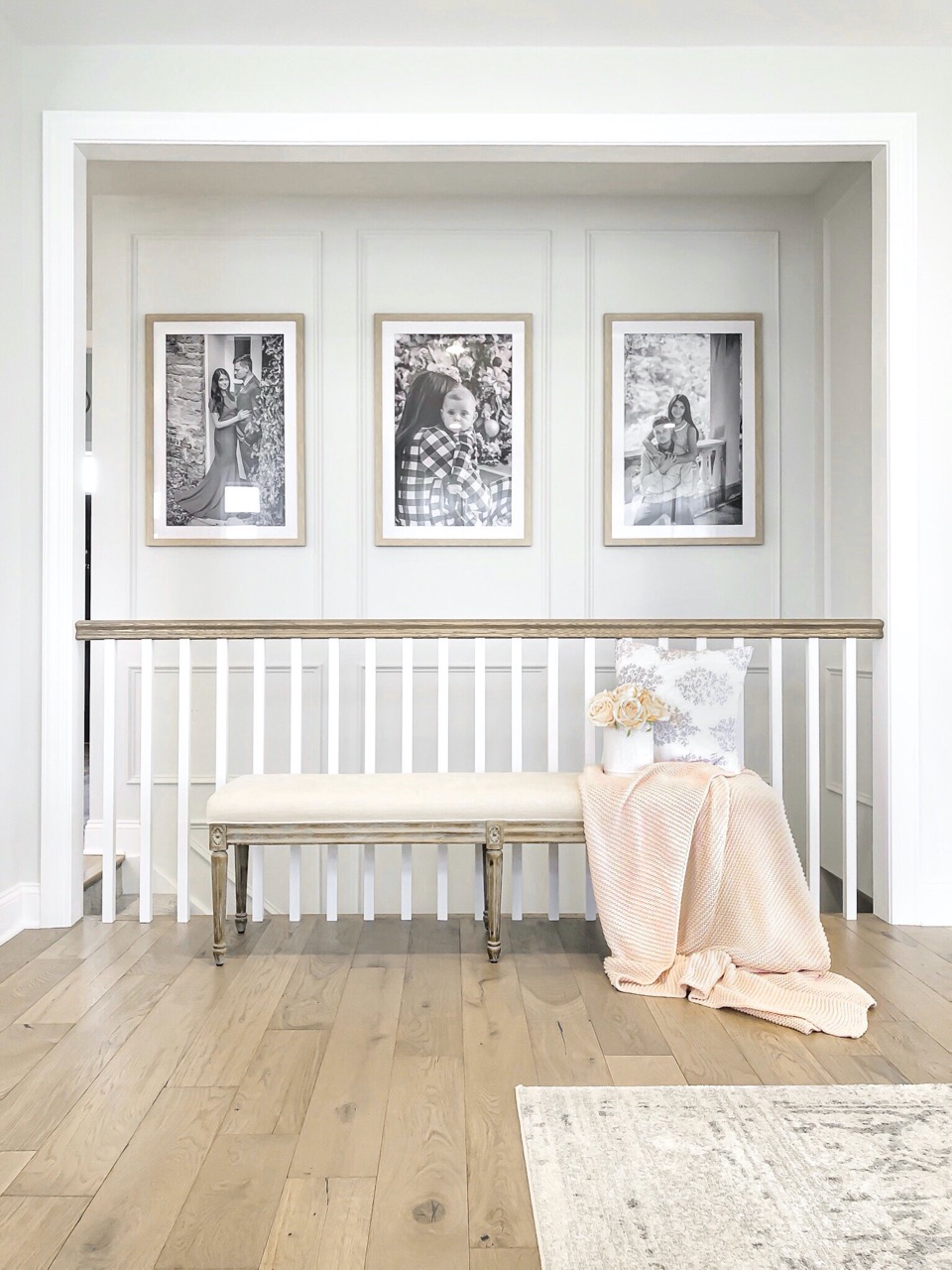The image captures an interior view from the upper floor of a home. The focal point of the scene is a set of gray-colored wooden stairs, partially visible at the top. In front of the stairs stands a gray railing with white spindles, leading to an archway that provides a glimpse of the stairwell area, which is painted white. 

Hanging on the white wall are three black-and-white artistic photographs, each enclosed in gray frames. The photographs depict: a man and a woman on the left, a woman holding a baby in the center, and a woman hugging a man from behind on the right. Below the photos, the floor is covered in gray wood.

Complementing the serene setting is a two-person bench with a cream-colored cushion and a gray frame, positioned comfortably to create a cozy atmosphere. The combination of neutral tones and personal photographs adds a touch of elegance and warmth to the home's decor.